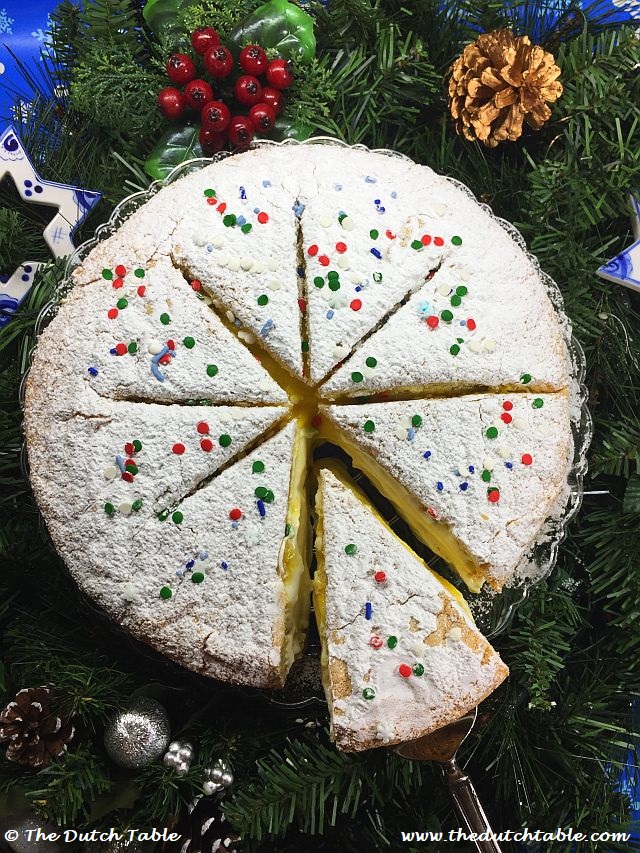The image showcases a festive Christmas cake covered in white powdered sugar, accented with red, green, and blue edible sprinkles. The cake, resembling a yellow pound cake, is sliced into eight pieces, creating a snowflake-like pattern when viewed from above. One slice is being lifted out with a silver cake spatula, revealing the cake's moist, custardy interior. The cake sits on a silver scalloped cake dish, surrounded by a decorative bed of evergreen pine branches, pine cones, and bright red berries, giving the appearance of a Christmas wreath. Additional festive elements, such as silver Christmas ornaments and ribbon, add to the holiday spirit. The image is vertically oriented, and in the lower left corner, there is a pine cone beside a silver Christmas ball and ribbon. The photo includes text in bold white script, with "© The Dutch Table" at the bottom left and "www.thedutchtable.com" at the bottom right.